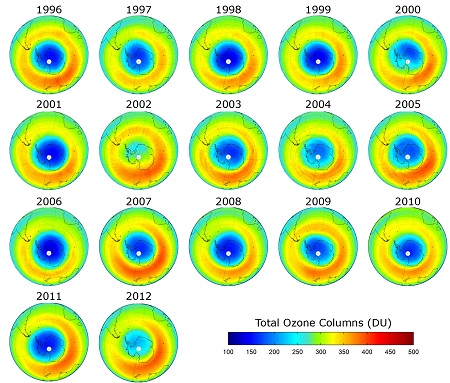This detailed colored diagram depicts the total ozone columns around Earth from 1996 to 2012. The diagram is organized into 17 circles, arranged in three rows of five and one row of two, each labeled sequentially by year. Each circle in the diagram contains concentric colored rings transitioning from green to blue, displaying ozone data as per the included legend. The legend at the bottom right, titled "Total Ozone Columns (DU)," uses a spectrum from blue to red to indicate ozone levels, ranging from 100 DU (dark blue) to 500 DU (dark red). The majority of the circles feature dark blue centers, with the exceptions of 2002 and 2012, which have light blue centers. Surrounding the blue centers, the circles exhibit colors transitioning from orange to yellow, eventually reaching light green at the edges. The colors within the circles reflect the values on the legend, showing the concentration of ozone from the outer green/light blue rings to the dark blue centers.